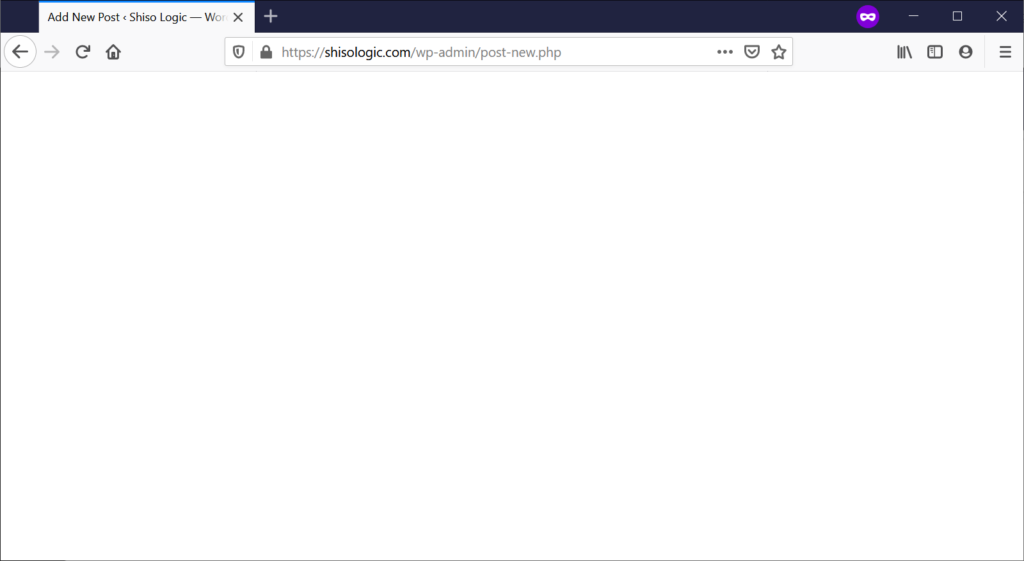**Detailed Caption:**

The image depicts a web page with a dark blue theme, viewed in a Firefox browser rather than Google Chrome. The URL displayed in the address bar reads "she's so logic." The background of the web page itself is white, while the top part of the browser window, including the minimize, maximize, and close buttons, is colored dark blue, aligning with the theme. Additionally, a circular purple icon with glasses is visible, suggesting that this may be Firefox's version of incognito mode. The web page features an option labeled "Add New Post." Overall, the layout is simple and does not include other significant elements.